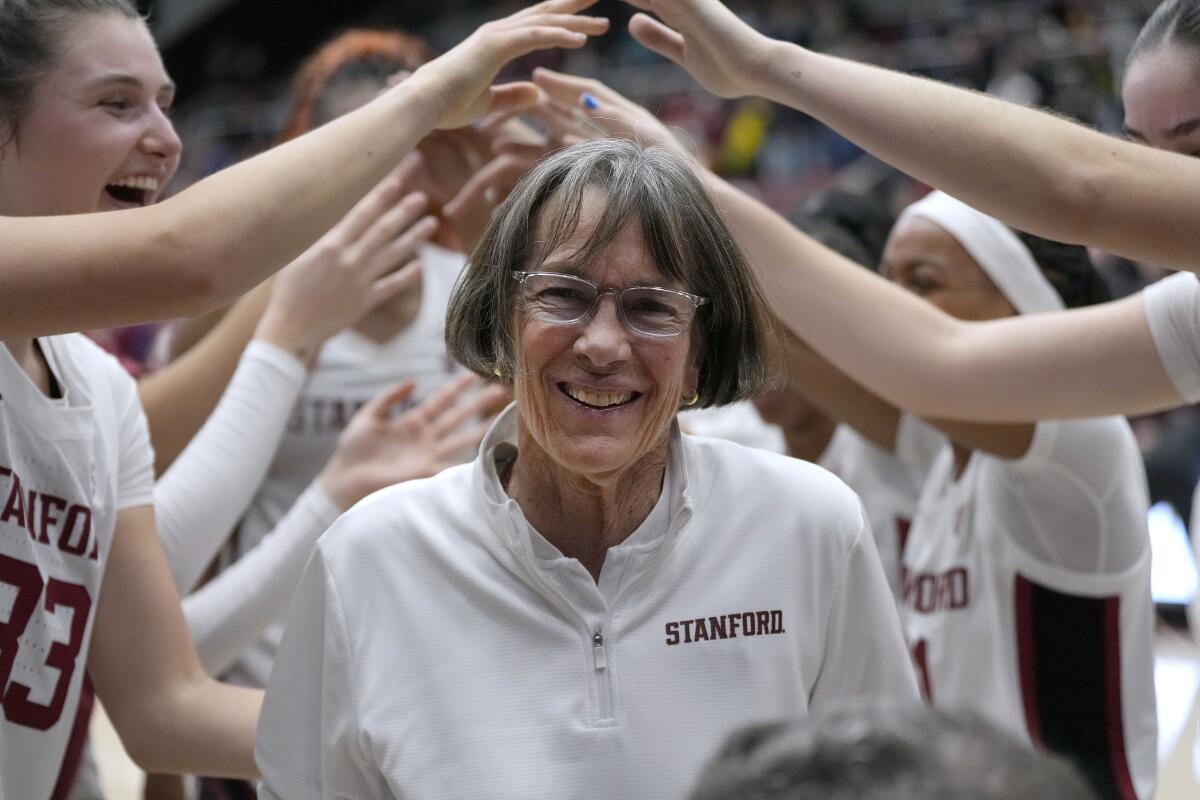In the center of this vibrant photograph is an older woman with short gray hair, sporting clear-rimmed glasses and a white quarter-zip jacket with "Stanford" emblazoned on the upper right part of her chest. Her beaming smile suggests her joy and pride as she stands amidst a celebratory scene. Surrounding her are enthusiastic college-aged female basketball players, all donning white jerseys with "Stanford" and their individual numbers. The players have their arms raised, creating an arch or tunnel that frames the woman, reminiscent of celebratory passageways often seen in jubilant moments. The camaraderie and happiness are palpable, with players smiling and laughing as they honor the central figure, who is likely their esteemed coach. The background subtly hints at the larger crowd in a stadium, purposefully blurred to keep the focus on this heartwarming moment of celebration and unity. The dynamic and joyful energy captured in this image highlights a special, celebratory moment for the Stanford women's basketball team and their dedicated coach.